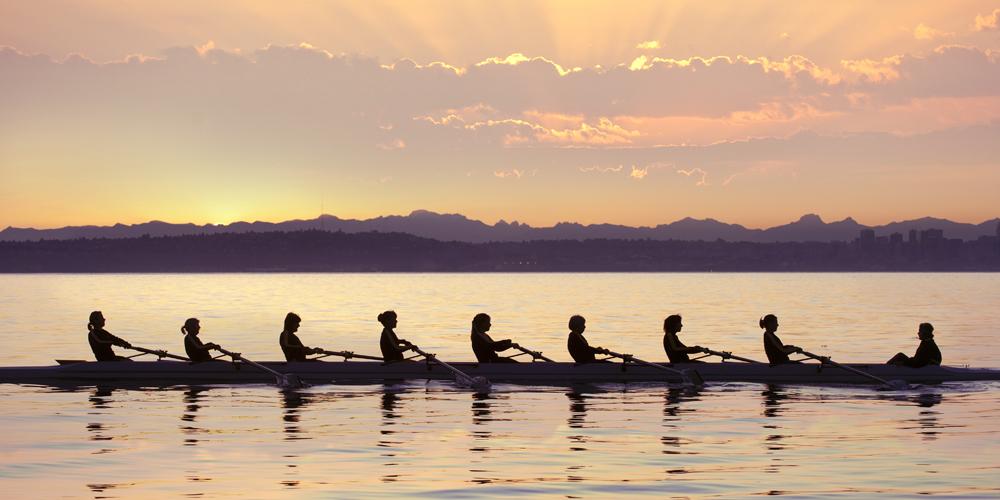The photograph captures a serene yet dynamic scene of a competitive rowing team set against the rich hues of a sunset. It presents a side view of a longboat in motion, with eight rowers silhouetted against the calm, reflective waters. Positioned on the right side of the image, a coach faces left, observing the rowers who are aligned from the center to the left, steadily propelling the boat forward with synchronized strokes. The sun, gently setting below the horizon, casts a peachy-pink and yellow glow across the sky, its rays piercing through the scattered clouds. In the hazy distance, silhouettes of tree-covered hills and distant mountains enhance the peaceful ambiance. The water mirrors the glowing sky, creating a harmonious interplay of light and shadow. The scene captures a perfect balance between human effort and natural tranquility.